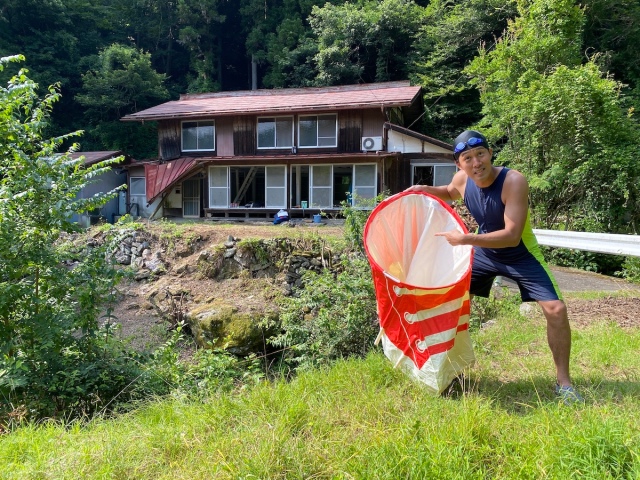In this detailed outdoor photograph, an Asian man, possibly a YouTuber, is captured goofing around. He stands on a piece of hilly terrain in front of a modern, two-story wooden house with numerous windows, nestled within a lush, green forest. The house appears brown, contrasting with the vibrant greenery. In front of the house, there's a steep ravine, possibly with a stream running through it, and some rocky landscape.

The man, dressed in a blue tank top and blue-green shorts, accessorized with swimming goggles and a swimming cap, exudes a playful vibe. He is holding a large, presumably new, sneaker with a red and white net-like design and pointing inside the bag with his left arm, directing attention to it. His expression is one of surprise or playful challenge, looking straight at the camera with an egging-on look. The sun is shining, adding brightness to the scene, and the backyard features tall, unkempt grass and a few bushes. The entire setting is vibrant and lively, capturing a spontaneous and fun moment.